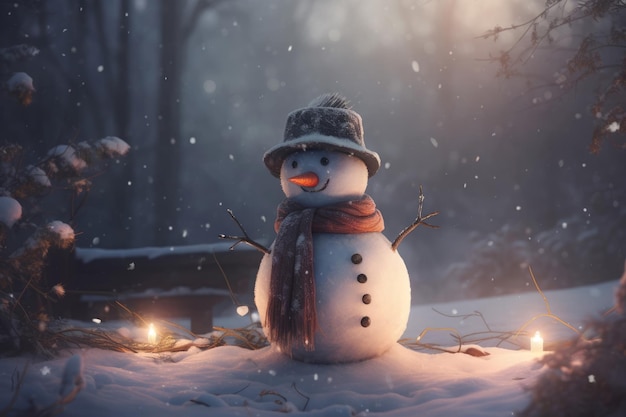In a scene reminiscent of Disney's live-action animations, the image portrays a picturesque, snowy landscape. Bare, brown branches adorned with a gentle layer of snow frame the scene, stretching across both sides of the visual. The ground is blanketed in a pristine, white carpet of snow. Adding a touch of warmth and enchantment, small, glowing lights or perhaps candles illuminate the lower corners of the image.

At the center of this enchanted winter wonderland stands a charming snowman. Constructed from two large snowballs, the snowman features a plump lower body with four round, black buttons prominently displayed. Wrapped around its neck is a scarf, which appears to be either red or brown, adding a splash of color to the scene. The snowman's arms are fashioned from slender twigs, giving it a friendly and welcoming stance.

Its head, smaller and perfectly spherical, boasts two black circles for eyes and a simple cavity where its nose would be. A black line curves into a cheerful smile, further enhancing its amiable demeanor. Atop its head rests a black hat, sprinkled with a delicate dusting of snow, completing the festive and heartwarming portrait set against a softly falling snow.